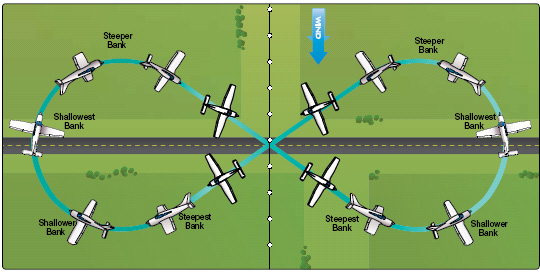This image is a detailed instructional graphic designed for pilots, illustrating a figure-eight maneuver. The top-down view showcases a cartoon depiction of a green landscape, divided into four sections with a central road featuring a divided yellow line running horizontally. Above the landscape, an airplane is depicted following the figure-eight path, highlighting different banking angles essential for the maneuver. Throughout the path, labels such as "shallowest bank" and "steeper bank" are strategically placed, emphasizing the transition in bank angles at various points of the figure eight. Two annotations, "steepest bank" and "shallowest bank" appear both at the top and bottom of the figure eight, attesting to the different stages of the maneuver. Additionally, in the right-hand upper corner, there's a label noting "steeper bank." The plane, represented in a white and black cartoon style, traces the turquoise outline of the figure eight on the green background, which is interspersed with darker green areas symbolizing bushes. A distinct black line with white circles runs vertically, and a blue arrow labeled "W1ND" adds to the instructional elements of the graphic.